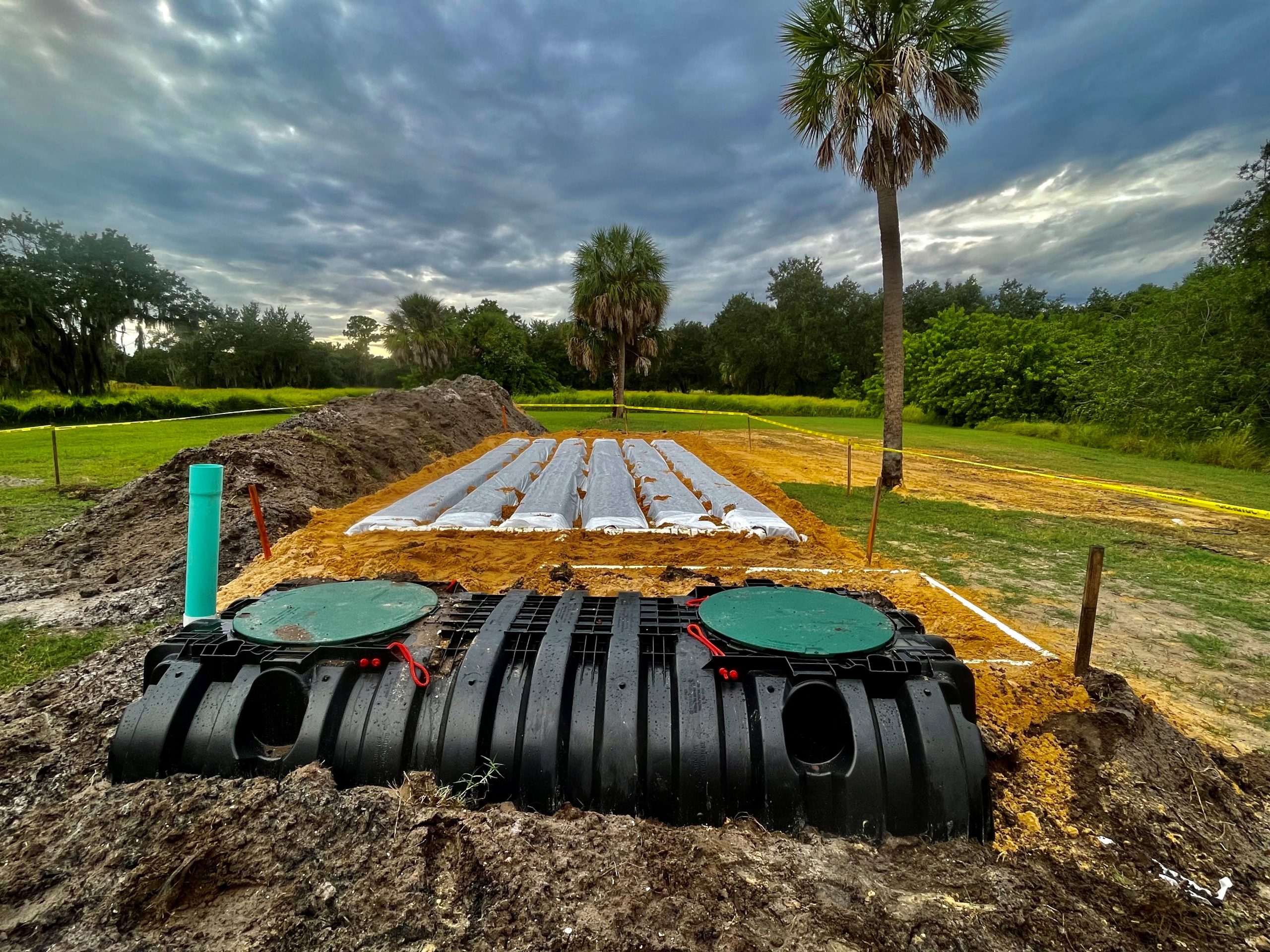In this photograph taken in a garden under a gray, overcast sky with pockets of light peeking through, a variety of lush green vegetation is showcased. In the background, a row of green trees lines the horizon, while a couple of tropical-looking palm trees stand solitary in the mid-ground. The foreground features a mix of green and yellow grass, with a section of yellowed grass containing long white strips whose purpose is unclear. Adjacent to this yellowed grass is a large pile of soil. Prominently in the foreground lies a piece of black cylindrical equipment with green pads on either end, marked with red and turquoise wires, possibly a farming tool. The scene includes a raised mound covered with what appears to be rows of crops, sectioned off with tape for containment. This detailed and purposeful setting captures both the beauty and functionality of the garden on a cloudy day.